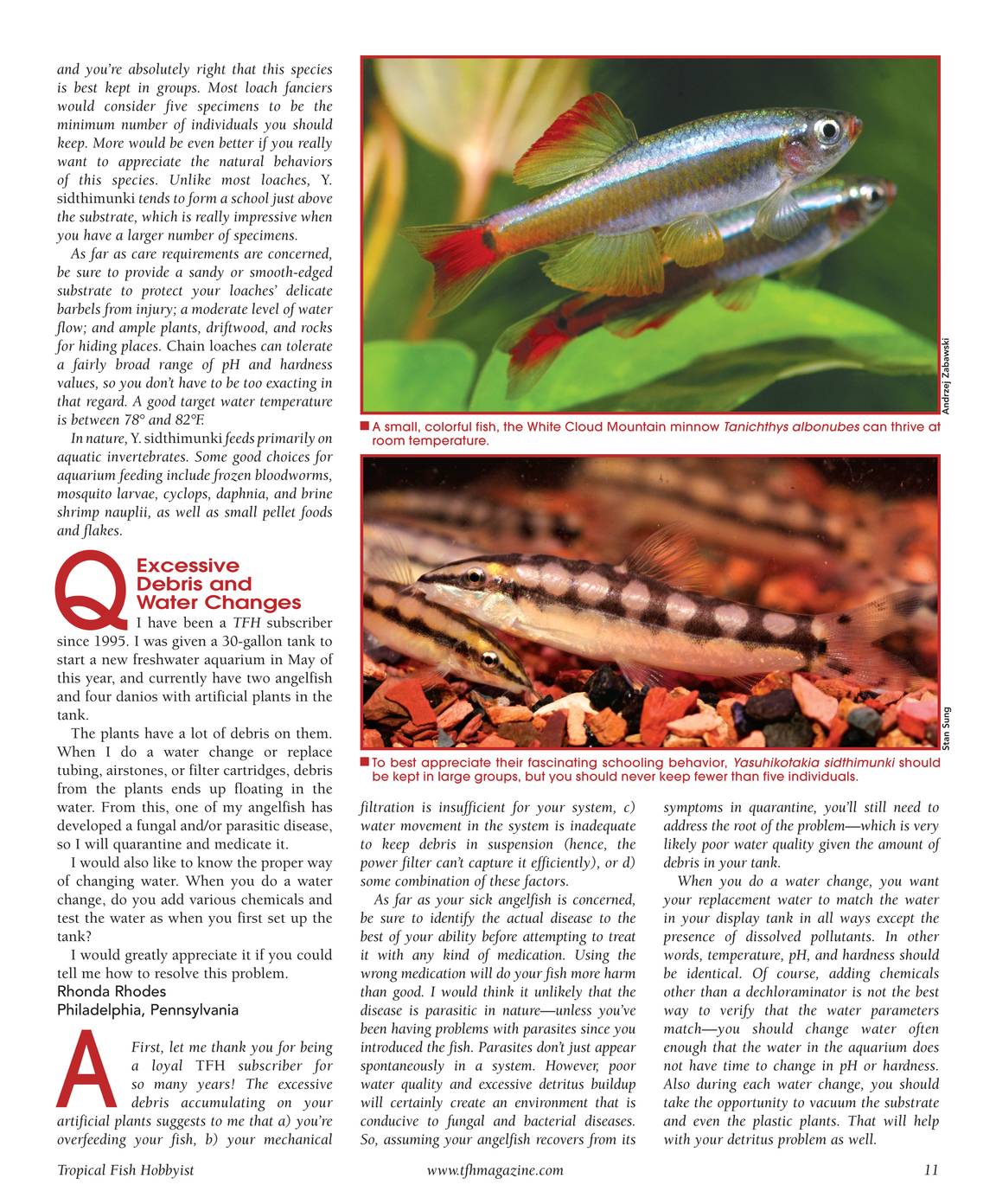This image appears to be a page from a scientific magazine or textbook, formatted similarly to a newspaper article. The page is primarily vertical in orientation and features two main sections with red headings titled "Excessive Debris and Water Changes." The text beneath the headings is black on a white background and includes a large "Q" and "A" representing a question and answer format.

In the upper right corner, there is a colorized image of two small, slender, and silver fish with green and red fins swimming in a tank adorned with green plants and leaves. This image is captioned: "A small colorful fish, the White Cloud Mountain Minnow, Tanichthys albonubes, can thrive at room temperature."

The second image below depicts a different type of fish, displaying darker and lighter tones with silver spots, situated at the bottom of an aquarium, among small rocks. The caption reads: "To best appreciate the fascinating schooling behavior, Yasuhikotakia sidthimunki should be kept in large groups, but you should never keep fewer than five individuals."